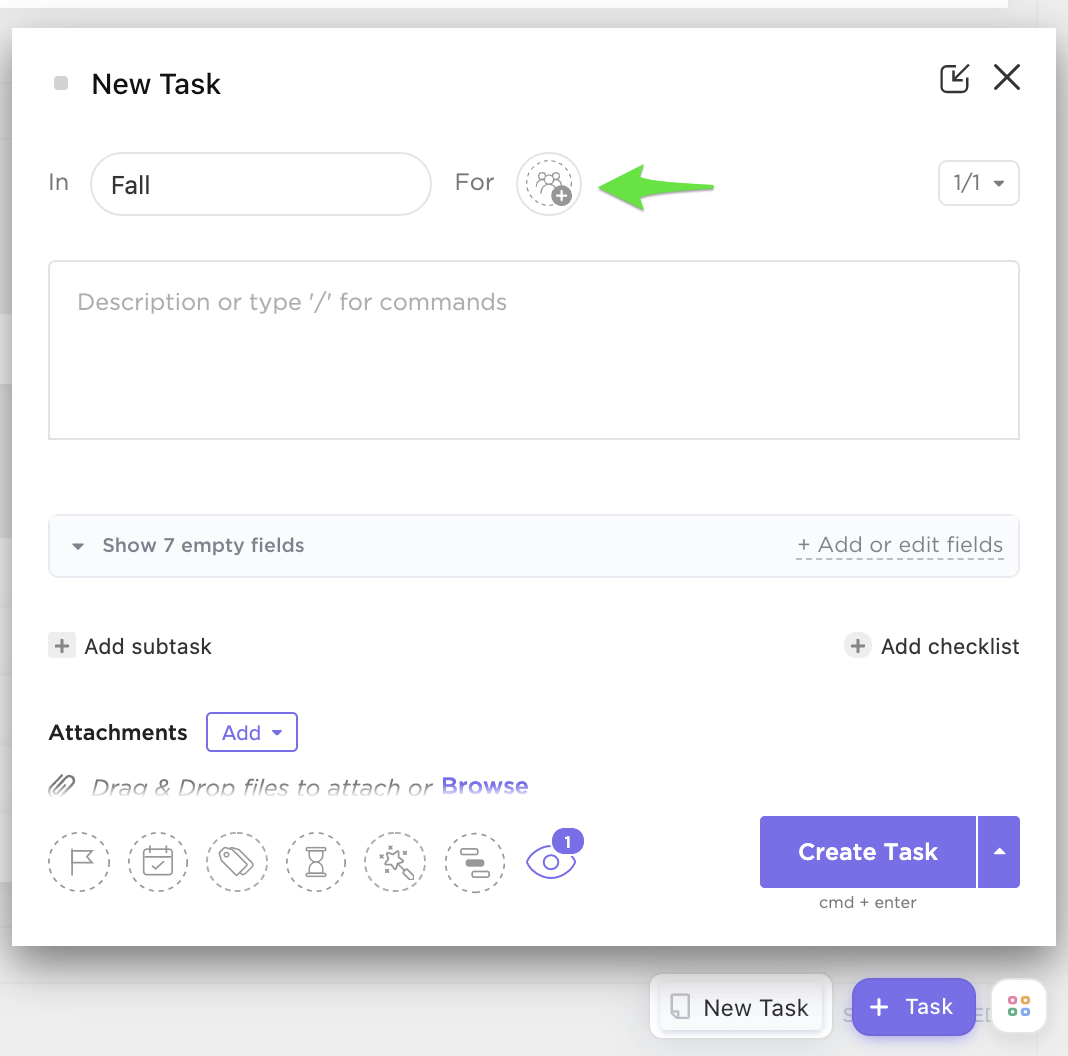The image is a screenshot from a task management application, showcasing a pop-up window that superimposes the main interface. The underlying interface is slightly darkened, suggesting that the pop-up was triggered by an action on the main screen. The pop-up features a white background with a purple color scheme for its buttons and notifications.

At the top of the pop-up, the title "New Task" is prominently displayed, flanked by a close button (an 'X') and a minimize button (a square with a downward-left facing arrow). 

Below the title, the pop-up contains a labeled input field: "In Fall", signifying that the task is designated for the fall season. Adjacent to this section is a label that reads "For". Next to this, there is an icon featuring three stick figures and a plus sign, indicating the option to add contacts who can view the task. 

Notably, a green arrow has been overlaid on the screenshot, pointing directly at the icon for adding contacts, emphasizing this particular feature for the viewer.